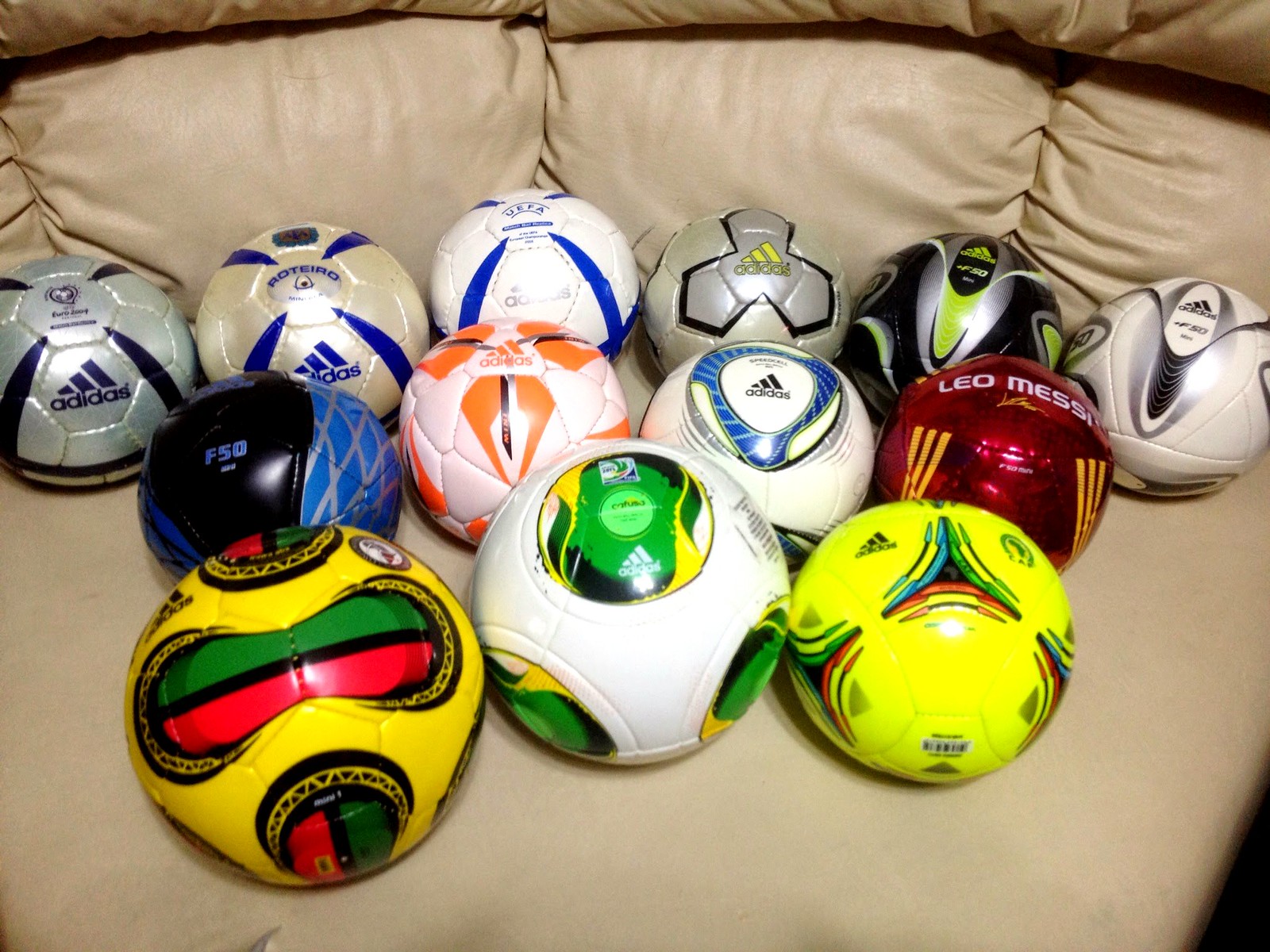The image is a detailed color photograph showcasing a light beige leather or pleather sofa, distinctive for its ruched back that forms pillowy shapes and a smooth flat seat. The sofa's back is textured, creating pillow-like forms, while its seat holds an array of 13 soccer balls arranged in a diminishing sequence of rows from the back to the front.

Along the sofa's backrest sits a row of 6 soccer balls: 
1. A silver ball with dark stripes and the Adidas logo.
2. A white and blue ball, also Adidas.
3. Another white and blue Adidas ball with a brighter hue.
4. A silver ball with black markings and a yellow logo by Adidas.
5. A lime green and black ball.
6. A white ball featuring op-art designs.

In the middle row, 4 soccer balls are aligned:
1. The F50 Adidas ball, characterized by blue and silver netted stripes.
2. An orange and white Adidas ball.
3. Another white and blue Adidas ball with a unique design.
4. A metallic red ball with yellow stripes, branded Leo Messi.

The front row of 3 soccer balls includes:
1. A ball with Jamaican colors: yellow, green, red, and black.
2. A white ball with round panels in light green and bright yellow.
3. A super bright yellow ball with triangular designs.

All the soccer balls, of various colors and designs, are prominently marked with the Adidas logo, signifying their brand consistency despite their diverse appearances.